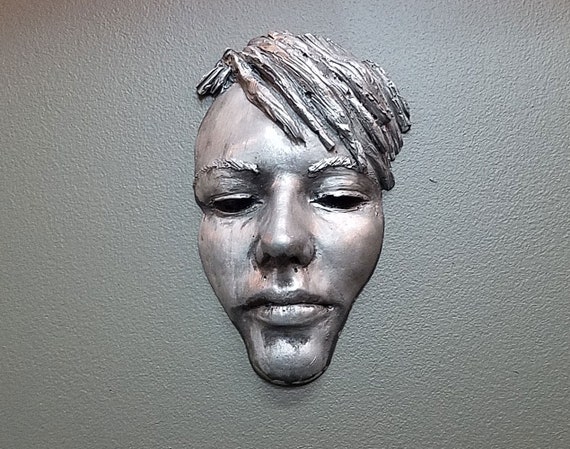The image portrays an intricately detailed decorative mask mounted on a textured, light gray wall. Designed to resemble the face of a human male, the mask features exaggerated, sculptural elements, giving it a striking and surreal appearance. Its most notable attributes include a very long, thin chin, large lips stretching across the entire face, prominent hollowed-out cheeks, and black holes replacing the eyes, accentuating its expressionless demeanor. The mask also includes a large, prominent nose and pronounced bushy eyebrows. Topping off the detailed features, the mask has dreadlocks sweeping to the right of the image, adding to its dramatic flair. Crafted to appear as if forged from metal, the entire mask is a striking silver, enhancing its artistic and decorative essence.